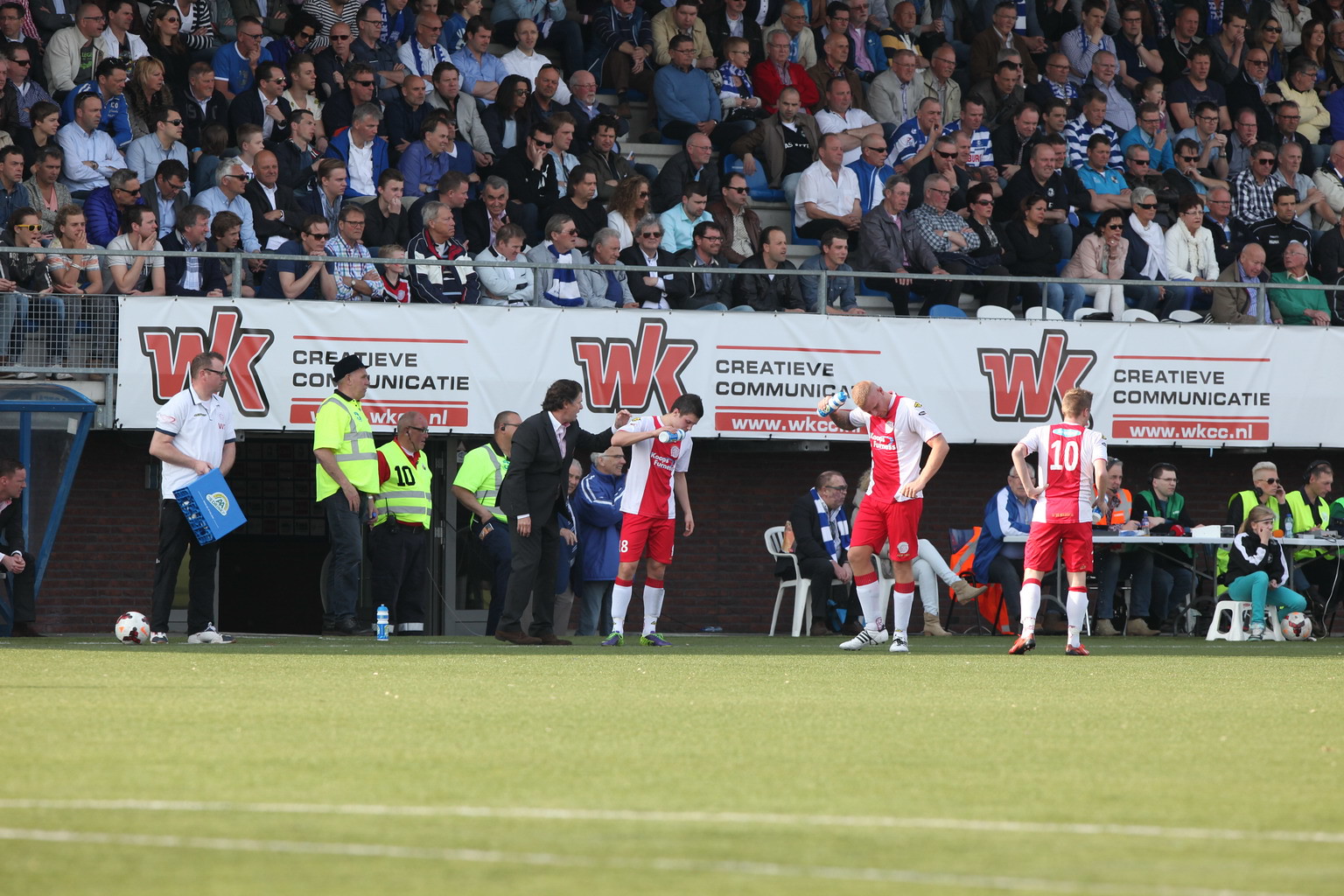The image captures a detailed scene at a soccer game, focusing on the sidelines. Three players from the same team are centrally featured, donning white jerseys with a red stripe down the middle, red shorts, and white socks with red accents. One player's jersey number, 10, is visible. To their left, there are several officiants and support staff, some in neon yellow vests and one in a white polo shirt. A coach or owner in a business suit can be seen yelling at a player. The scene is lively with a sponsor banner from WK Creative Communications (www.wccc.nl) stretching horizontally across the top third of the image. In the background, a stadium filled with fans avidly watching the match is visible. A man holding a blue kit suggests someone might have been injured. To the right, a group of people is seated at tables. The primary colors in the image are red, blue, light yellow, and green, highlighted against the green pitch and overall scene, which exhibits photographic representational realism.